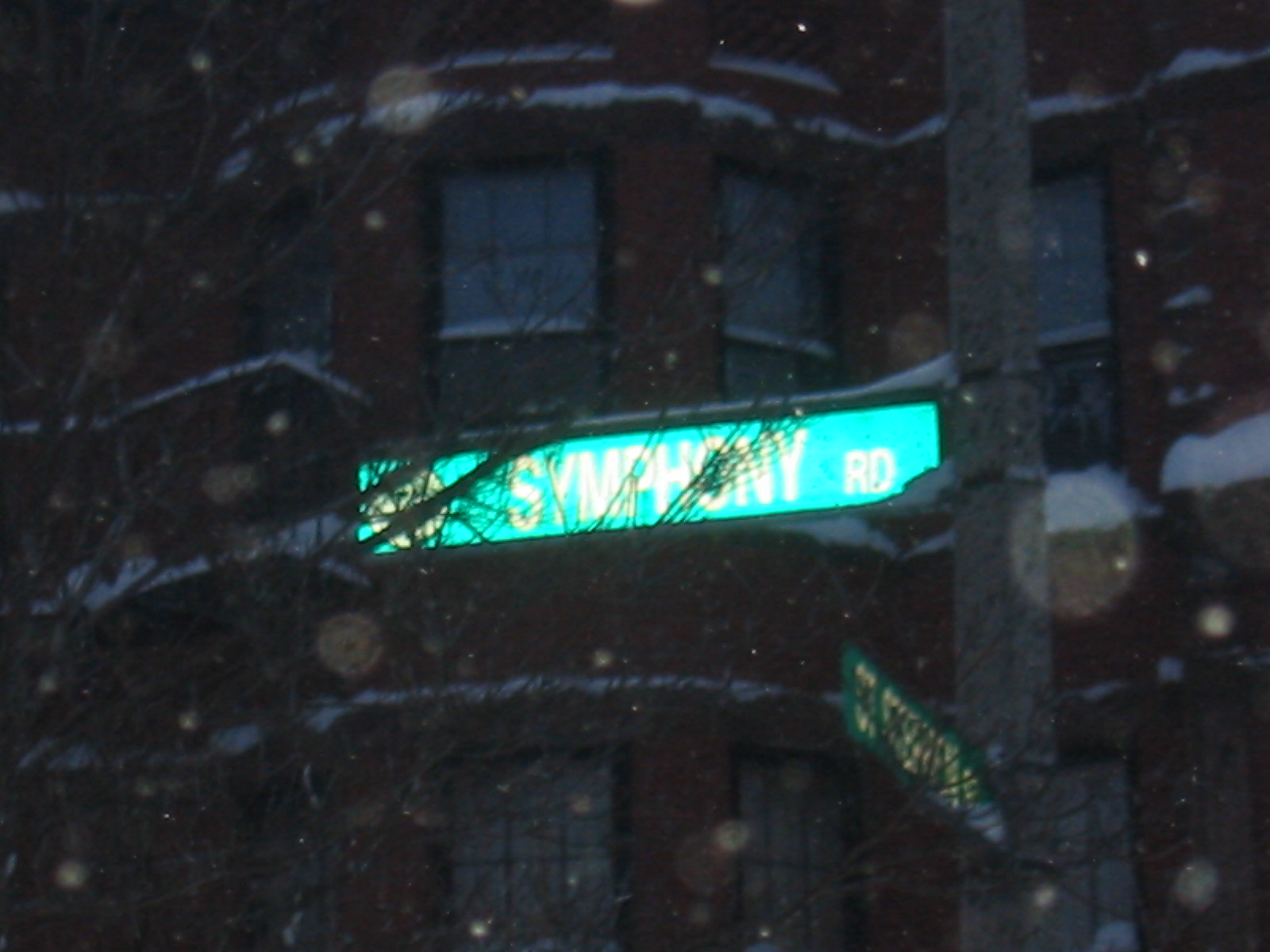A green street sign reading "Symphony Road" stands prominently against a complex background. The sign, made of highly reflective material, features crisp white lettering. Snow particles float gently in the air, creating a serene atmosphere. The sign is affixed to a sturdy gray pole, partially obscured by bare tree branches. In the background, a venerable brick building rises to three stories or more. This structure boasts a series of windows, each adorned with tightly closed white blinds, hinting at a story of privacy and introspection. The scene invites viewers to imagine the warmth of sunlight should those blinds be drawn open.